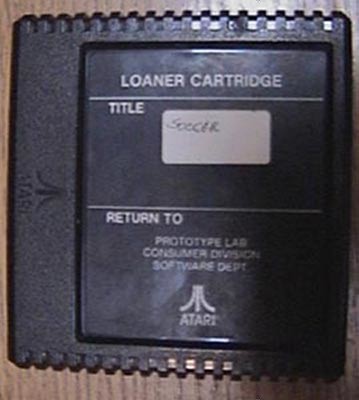This detailed image portrays a vintage Atari video game cartridge placed on a wooden tabletop with varying shades of brown, reminiscent of a desk. The primary feature of the photo is the black, rectangular cartridge which prominently displays the label "LOANER CARTRIDGE" in white, capitalized text at the top right. Below this, within a white rectangular box, is the handwritten word "Soccer". The label further includes a line that reads "Return to Prototype Lab, Consumer Division, Software Department, Atari" emphasizing its prototype status. The cartridge itself has a distinctive design with rough, tooth-like edges at the top and bottom, adding a unique texture to its appearance.